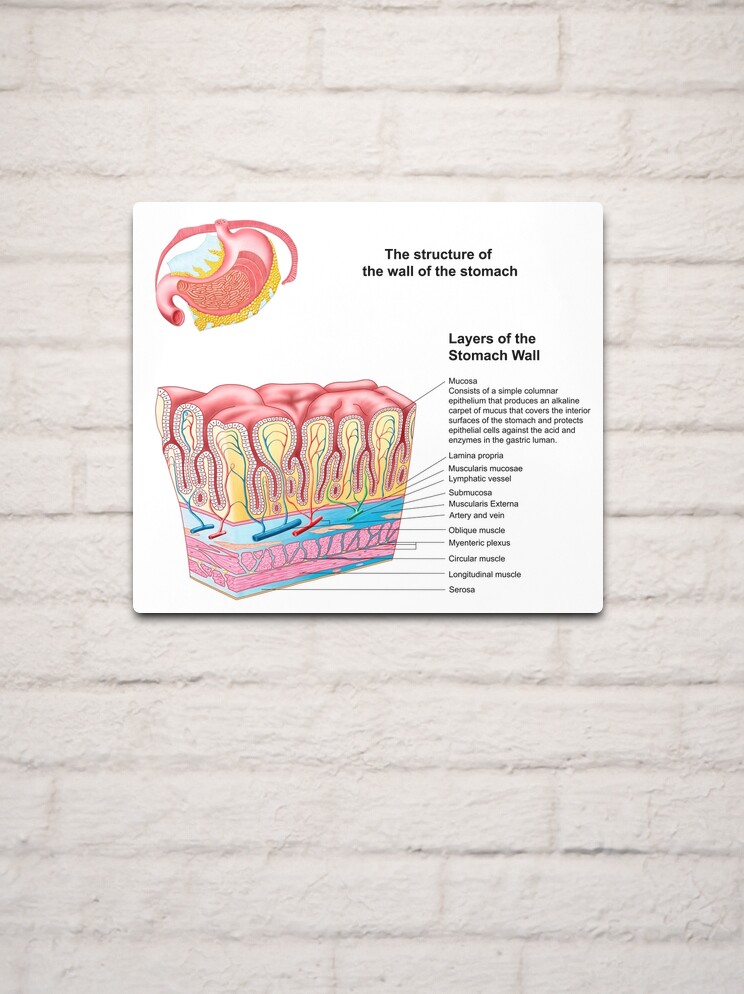This is a small, square informational graphic titled "The Structure of the Wall of the Stomach," displayed on a white or off-white brick wall. The top right of the poster features the title in small black letters. On the left side of the poster, there are two images in color. The top-left image is a depiction of the stomach, showing its pink-colored interior. Below it, the bottom-left graphic is a detailed, rectangular, and three-dimensional illustration that presents the different layers of the internal wall of the stomach. This graphic uses a color scheme including blue, red, yellow, pink, and blue at the bottom. To the right of these images, the poster has black text titled "Layers of the Stomach Wall," with arrows pointing to each respective layer in the illustration, providing clear and detailed labels.